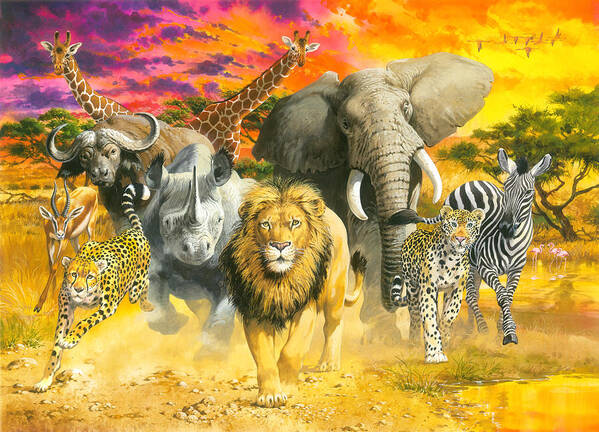This vibrant digital portrayal of an African savannah scene features a diverse assembly of wildlife seemingly charging towards the viewer. At the heart of this animated tableau stands a majestic lion, its golden coat and black mane drawing the eye. Just to the lion's left, a formidable gray rhinoceros holds its ground slightly behind the big cat, while a powerful gray elephant trails further back to the lion's right. Flanking these central figures are two lithe leopards, one prowling near the rhinoceros and the other shadowing the elephant. Further out to the right, a striped zebra gallops, and to the left of the rhinoceros, a tan buffalo is depicted with two giraffe heads peeking out just behind it, adding height and elegance to the grouping. On the far left, a yellow emu and an antelope can be spotted, completing this bustling menagerie.

The terrain beneath the animals is a striking mix of bright yellow and orange, punctuated with hints of green. Sparse but vivid greenery and small, bonsai-like trees dot the landscape, indicative of the savannah's characteristic flora. The sky above transitions from deep purples and pinks on the left to warm yellows and oranges on the right, suggestive of either dawn or dusk. High in this colorful sky, simple, undetailed forms of birds—perhaps ducks or pelicans—are seen flying, adding life to the horizon. In the midst of this dynamic scene is a small body of water to the right, reflecting the sky’s brilliant hues and completing this detailed, energetic panorama of African wildlife in motion.